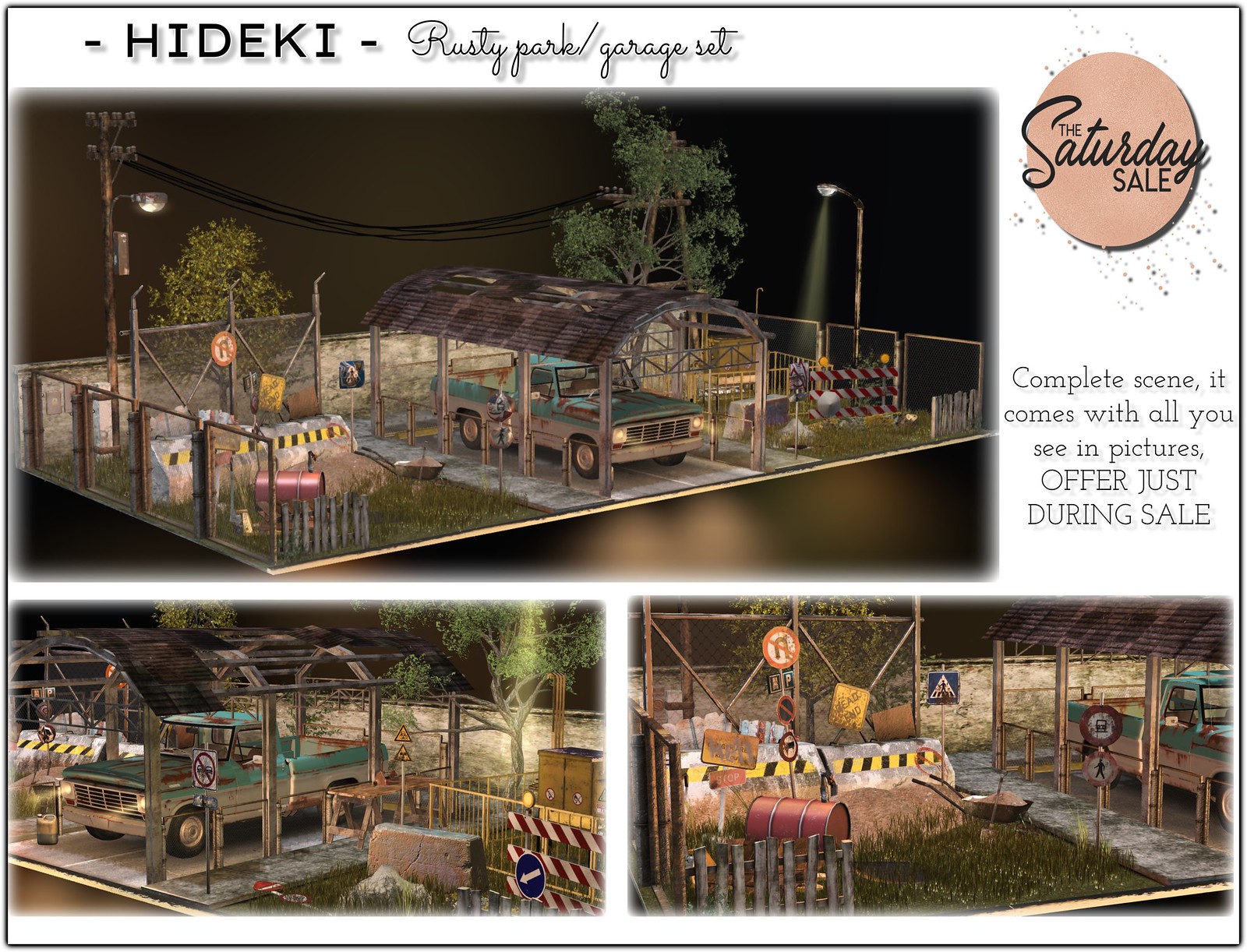The image is a detailed collage of three digital 3D renderings depicting an abandoned garage scene, evocative of a dystopian, post-apocalyptic setting. Central to the scene is a dilapidated, rusty pickup truck, predominantly light blue and white, situated under a heavily corroded outdoor cover. Surrounding the truck is a backdrop of broken concrete, dirt patches, and disheveled grass, giving the area a derelict appearance. Various elements such as construction barriers (including jersey barriers), chain-link fences topped with barbed wire, street lights, red barrels, and warning signs add to the chaotic, abandoned ambiance. At the top of the collage, in bold black text against a white background, it reads "Hideki Rusty Park Garage Set." On the upper right of the image, a brown circular logo for "The Saturday Sale" is displayed, accompanied by the text, "Complete Scene: It comes with all you see in pictures offered just during sale," indicating that the 3D artist offers this comprehensive scene for purchase during the sale.